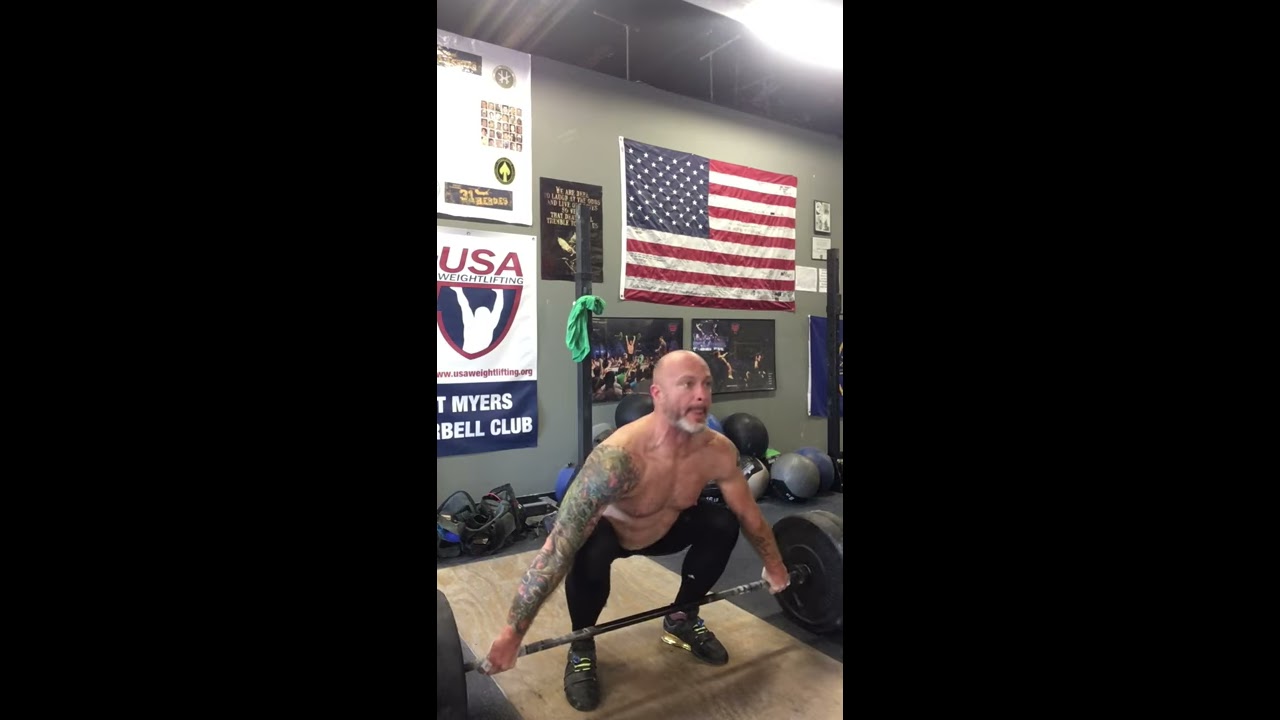In the image, a bald, shirtless man with a mix of dark gray and white facial hair, including a goatee, is poised in a squatting position, about to lift a barbell with large weights on each end. He is clad in black leggings and gray sneakers with yellow laces, standing on a tan mat within a gym that appears to be his own. His left arm, which is prominently tattooed in dark green hues, is visible as he prepares to lift. Behind him, a gray wall displays various items: on the upper right, an American flag; to the left, a black plaque with golden lettering; and further left, several posters. One poster features a figure lifting with "USA" and "Myers Bell Club" partially visible. Below this, there are more weights, gym equipment like medicine balls, and a duffel bag scattered around. The scene captures the intense, prepared moment before the lift in a well-equipped gym setting.